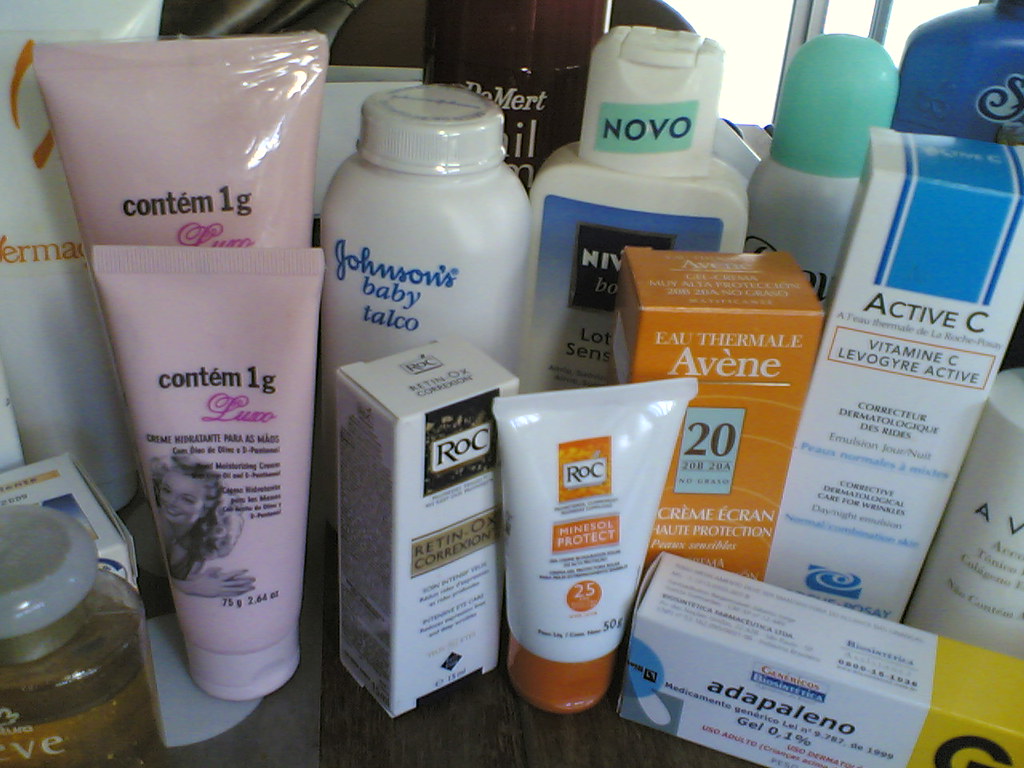In this detailed image, the edge of the table is barely visible due to the numerous items covering its surface. Starting from the left, there are multiple bottles, tubes, and boxes. On the far left, a gold-tinted liquid is visible inside a bottle with a white and gold lid. Next to this, there are two pink bottles labeled "Contine one gram," each featuring a woman's face. To the right of these pink bottles is an unopened container of Johnson's Baby Powder.

Further along, an ROC box is situated beside a white tube adorned with an orange label and an orange lid. Continuing to the right, there is a white bottle with a blue label, marked "Nova" across the lid. Below it, there is an orange box labeled "Vain." Beside this, a three-fourths white and one-fourth yellow box labeled "Adaptalino" stands out.

Behind the white and yellow box, there is an "Active C" box, which is predominantly white with blue accents. Adjacent to it, a white bottle with a brown body and a round green lid can be seen. Finally, partially obscured, a white bottle marked with a single visible "B" rests behind the yellow Adaptalino box. This detailed array of items presents a cluttered yet intriguing composition on the table.